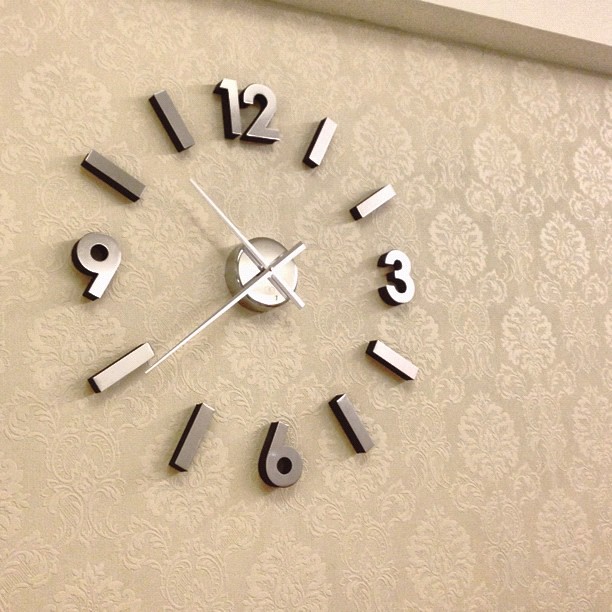The photograph showcases a minimalist wall clock featuring a modern design. Unlike conventional clocks with a rounded face, this clock consists of only the numerals 12, 3, 6, and 9, which appear to be a sleek silver color. These numbers are interspersed with minimalist hash marks indicating the other hours. At the center of the clock, a small, chrome-colored circle anchors the shiny chrome clock hands. The clock is mounted on a wall adorned with intricate, gray-and-white patterned wallpaper, adding a touch of elegance and sophistication to the overall aesthetic.